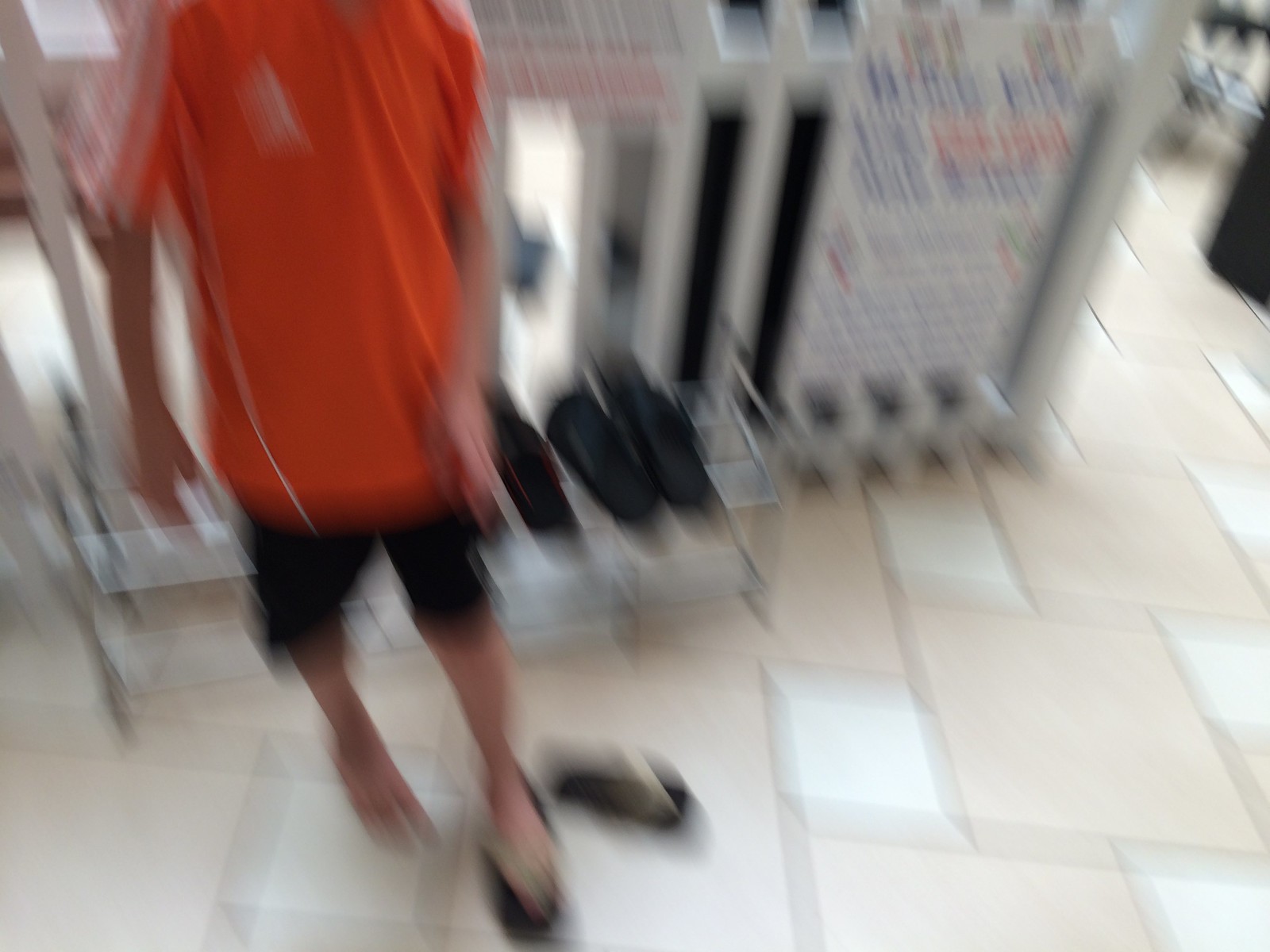The image is a very blurry photograph taken indoors, likely in a store based on the context. The photo captures a person from their shoulders to their feet, standing on the left side of the frame. This individual is wearing an orange t-shirt with some white accents, black shorts, and a single black flip-flop on their left foot, while the other flip-flop lies next to their bare right foot. They are standing on a tiled floor featuring a pattern of alternating tan and white tiles. Behind the person, there appears to be a rack displaying additional pairs of flip-flops, although the blurriness makes it difficult to discern details. There is also a sign with white and blue text that is illegible due to the camera movement, which creates up-and-down streaks throughout the image, further obscuring the background elements.